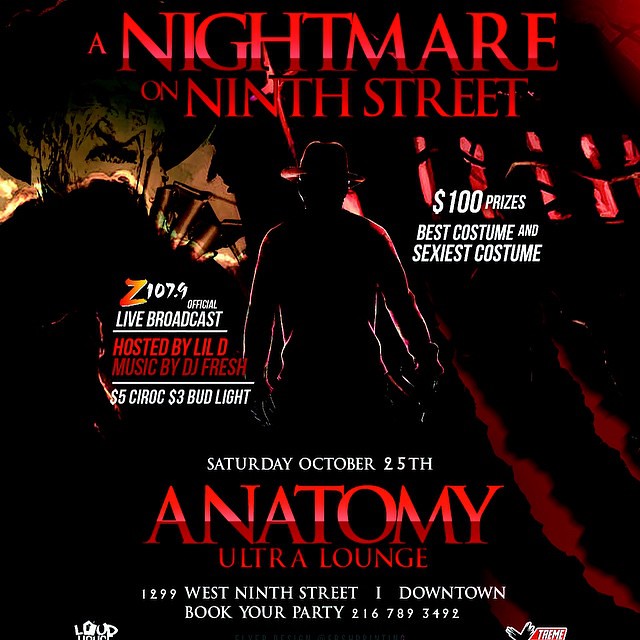The image is a square-shaped advertisement for an event at Anatomy Ultra Lounge titled "A Nightmare on 9th Street," prominently displayed at the top in red font. The dim, eerie background features the silhouette of Freddy Krueger, facing away while exuding a creepy, dark atmosphere. The ad features details in both red and white fonts. On the right, it announces "$100 prizes for best costume and sexiest costume." On the left, it reveals "Radio Station Z 107.9 official live broadcast hosted by Lil D, with music by DJ Fresh." Below this, it promotes "$5 Ciroc and $3 Bud Light," followed by "Saturday, October 25th" in bold text. At the bottom, the venue details are highlighted in red font: "Anatomy Ultra Lounge," and in white font: "1299 West 9th Street, Downtown. Book your party at 216-789-3492." The bottom also features icons for sponsors or DJs, though they are partially cut off.